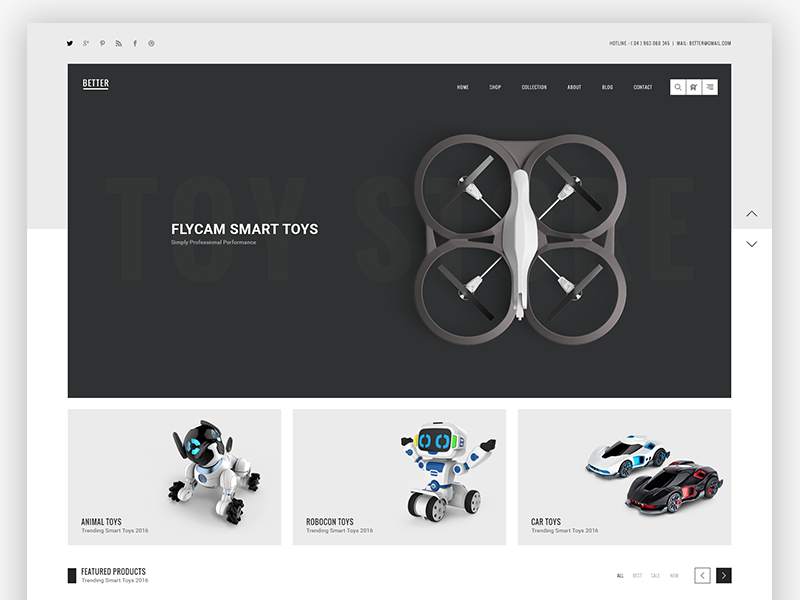The image is a screenshot from a website that can be divided into three main sections. At the very top, there's a social media bar to the left featuring icons for Twitter, Facebook, etc., and on the right, there’s a phone number and website link. Below this is a prominent black box occupying about two-thirds of the image. 

Inside the black box, in the top left corner, the word "BETTER" is displayed in gray font, contrasting against the black background. On the right side of this box is the main navigation menu in gray font, listing items such as Home, Shop, Collection, About, Blog, and Contact. Adjacent to these menu items are several buttons, including a discernible search button, with others that are unclear.

On the left side of this black box is an image of a quadcopter drone labeled "Flycam Smart Toys" with the text superimposed over it. Below this image, in lighter font, the words "Toy Store" are faintly visible.

Beneath the black box, there are three images showcasing different toy categories. The first image on the left displays "Animal Toys," featuring a robot that resembles an animal. The middle image, labeled "Robocon Toys," depicts a humanoid robot with a smiley face. The right image highlights "Car Toys," showing automated smart cars.

At the bottom left of the image is a button labeled "Featured Products," and on the bottom right, there are additional navigational controls.